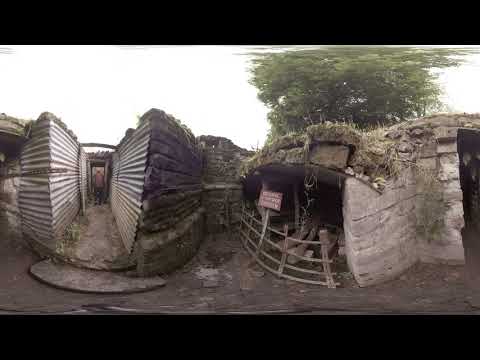This panoramic shot of an archaeological or historical site captures a series of dilapidated brick and concrete structures, possibly resembling World War I trenches or ancient ruins. The heavy distortion from the fisheye lens results in blown-out proportions and a thick black border at the top and bottom of the image. The structures, some with grass and moss-covered roofs, feature small alcoves and a mixture of dirt and paved pathways.

In the foreground, there is a notable brick enclosure with an indiscernible rusty red sign in the center, behind a rickety wooden fence. The middle ground reveals a metal-grated trench-like pathway with some vegetation growing in the cracks, where an individual clad in a rusty-colored shirt and jeans can be seen walking. The surroundings are enclosed by stone walls and concrete huts with small alcoves within.

A tall tree stands towards the back right of the image, enhancing the outdoor setting, which is marked by an overcast sky cast in a whitish hue. Overall, the scene exudes a worn, ancient ambiance with a mixture of natural elements and man-made remnants.